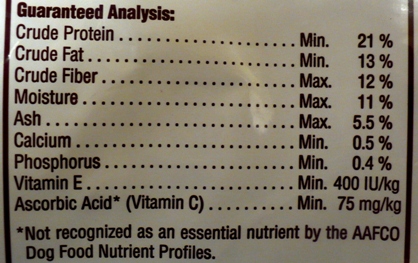The image displays the nutritional information section on the shiny packaging of a dog food product. The heading "Guaranteed Analysis" is prominently printed in bold black letters. Below this heading, there is a list of nutritional components: Crude Protein, Crude Fat, Crude Fiber, Moisture, Ash, Calcium, Phosphorus, Vitamin E, and Ascorbic Acid. Each of these terms is followed by dots leading to the word "MIN," which likely stands for "Minimum," and then a corresponding percentage value. At the bottom, there's an asterisk note stating, "Not Recognized as an Essential Nutrient by the AAFCO Dog Food Nutrient Profiles." The reflection of the camera's light is visible in the upper left corner, emphasizing the shiny nature of the package material.